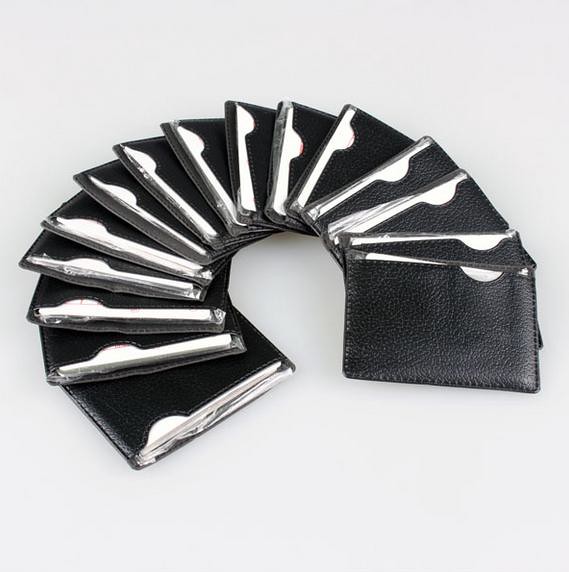The image displays an array of sleek, black leather card holders fanned out in a half-circle formation on a light gray surface. Each card holder, characterized by its slender and compact design, features a semi-circular cut-out that reveals a stack of white cards within. The texture of the leather is clearly visible, and the holders appear to be uniformly filled to a similar capacity, suggesting careful arrangement. The black and white aesthetic accentuates the fine details of the leather, while the consistent, thin profile of each holder indicates they are designed for minimalistic convenience. There are approximately 14 to 15 card holders in the image, perfectly laid out to emphasize their shape and craftsmanship.